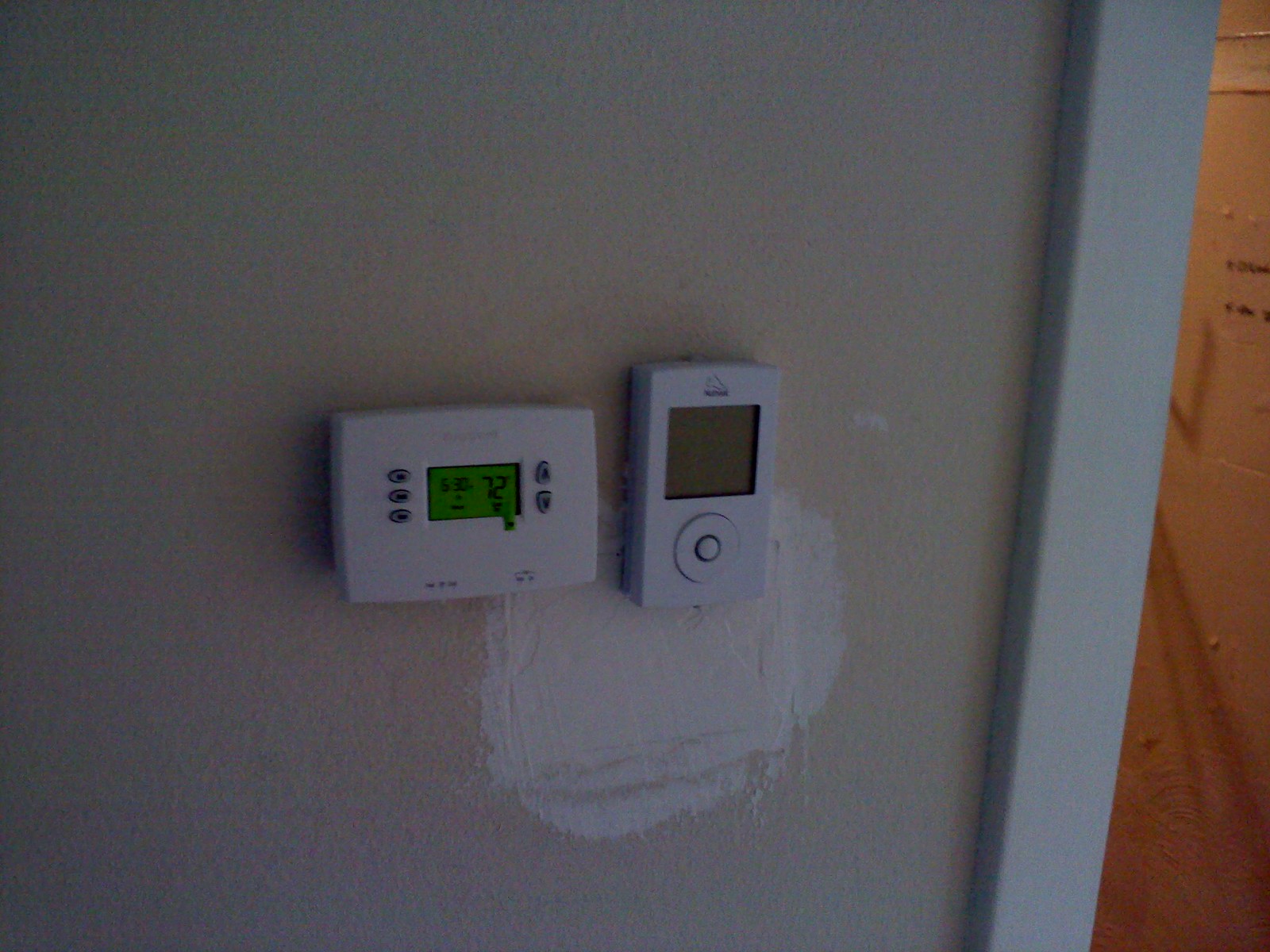The image depicts an off-white wall occupying approximately 75% of the left side of the frame. The wall appears to be patched in an area where a double-wide outlet or switch would typically be located, although the spackled area has not yet been sanded down. Mounted on this wall is a horizontal rectangular thermostat. The thermostat is off-white with a green screen displaying black text showing the temperature as 72 degrees. It features three buttons on the left and two buttons on the right. Adjacent to the thermostat, to its right, is a vertical gray device with a gray display, seemingly inactive, and a circular control wheel at the bottom that resembles an old iPod design.

To the right edge of the wall, there is a light blue trim framing an adjacent doorway. Through a narrow gap in the trim, part of a medium brown door is visible, adding a contrasting element to the otherwise neutral wall setup.